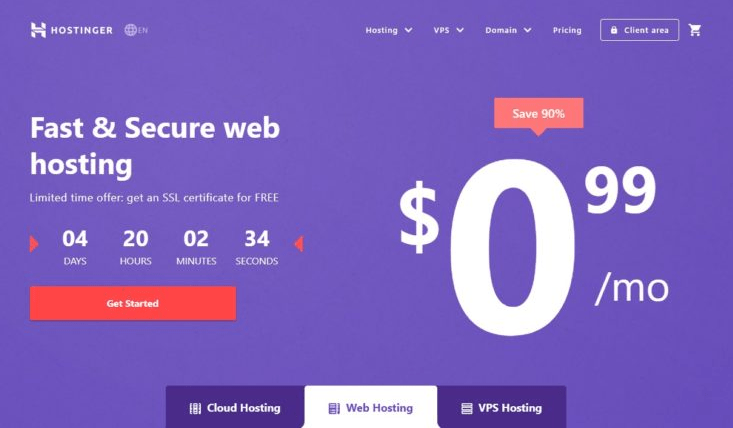The advertisement is a rectangle with an orchid-colored purple background. At the top-left corner, there is an icon with the text "Hostinger" beside a globe logo. Towards the center are menu options: "Hosting ↓", "VPS ↓", "Domain ↓", and "Pricing". Adjacent to these, there's a white-outlined rectangle featuring a lock icon labeled "Client Area", followed by a shopping cart icon.

Moving down the left side of the ad, the text "Fast and Secure Web Hosting" is displayed prominently, followed by the words "Hosting" on a new line. Below this, it states "Limited Time Offer: Get an SSL Certificate for FREE" with "FREE" in capital letters. Then, a countdown timer is shown with "04 Days," "20 Hours," "02 Minutes," and "34 Seconds" in white text, flanked by a forward and a backward arrow.

A red, clickable bar reading "Get Started" in white text is positioned below the timer. Below this, it displays "0.99 per month" in larger text, followed by an orange square thought bubble indicating "Save 90%."

At the bottom center of the ad are buttons for "Cloud Hosting," "Web Hosting" (highlighted as the current selection), and "VPS Hosting," all designed to be clickable.